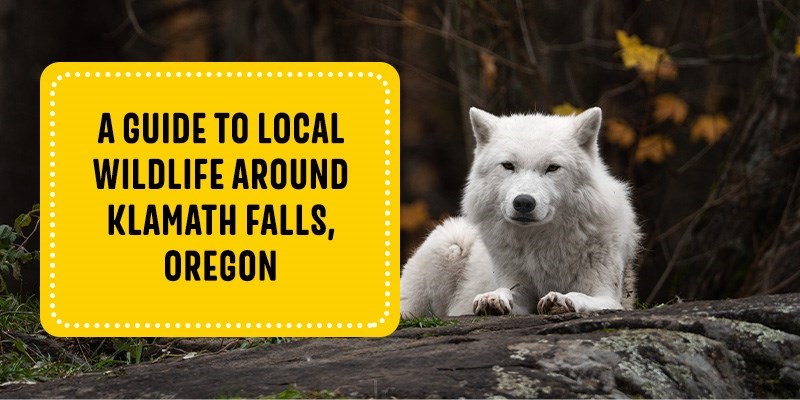The image is a realistic, horizontally-aligned photograph, likely serving as an advertisement or flyer. It features a striking, bright white wolf, possibly mistaken for a dog, that is the primary focus of the image. The wolf is lying down on a large, dark rock, with its front paws extending towards the camera and its black nose and eyes clearly visible. Its white ears stick up, contrasting against the dark, wintry forest background composed of bare trees, twigs, bushes, and occasional yellow leaves.

On the left side of the image, there is a prominent yellow rectangular text box with white polka dots around the edges. Inside, in black font, it reads: "A guide to local wildlife around Klamath Falls, Oregon." The overall palette of the image predominantly features dark browns and blacks typical of a forest in winter, which makes the well-lit, snow-white coat of the wolf stand out even more dramatically.